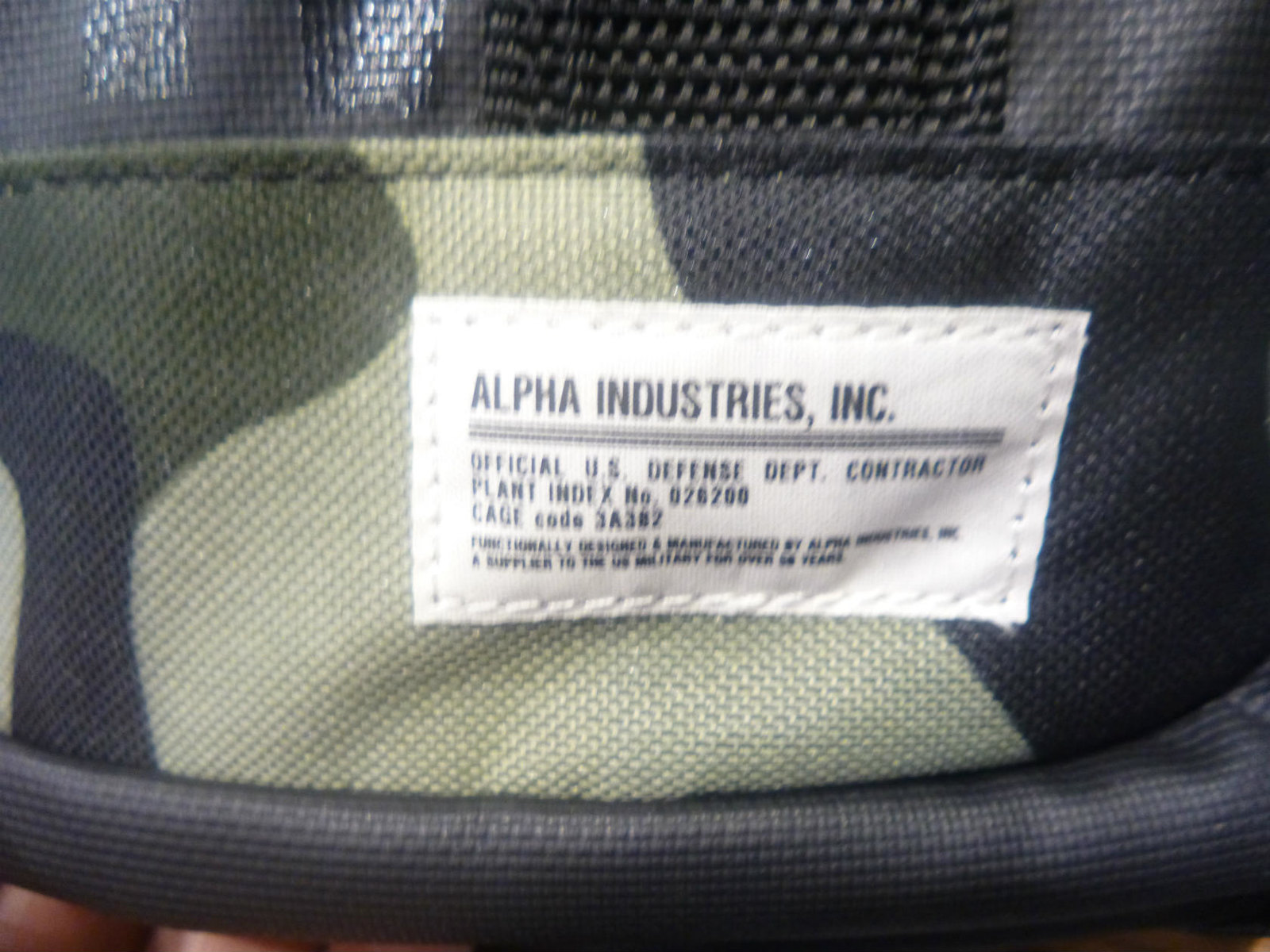This is a detailed photo showcasing the label inside a sturdy camo-colored bag made of thick material. The upper part of the bag features a cloth-like material coated with some kind of durable coating, providing additional protection and resilience. The bottom edge of the image is dominated by a prominent, thick, round hem that enhances the bag's robust construction. The label visible in the picture reads "Alpha Industries Incorporated" on the first two lines, followed by "Official U.S. Defense Department Contractor." It also includes additional information: "Plan Index Number 026200" and "CAGE Code 3A387." A hand is partially visible in the bottom left corner, holding the bag, and smaller words can be seen at the bottom of the label, though they are not fully legible in the image.